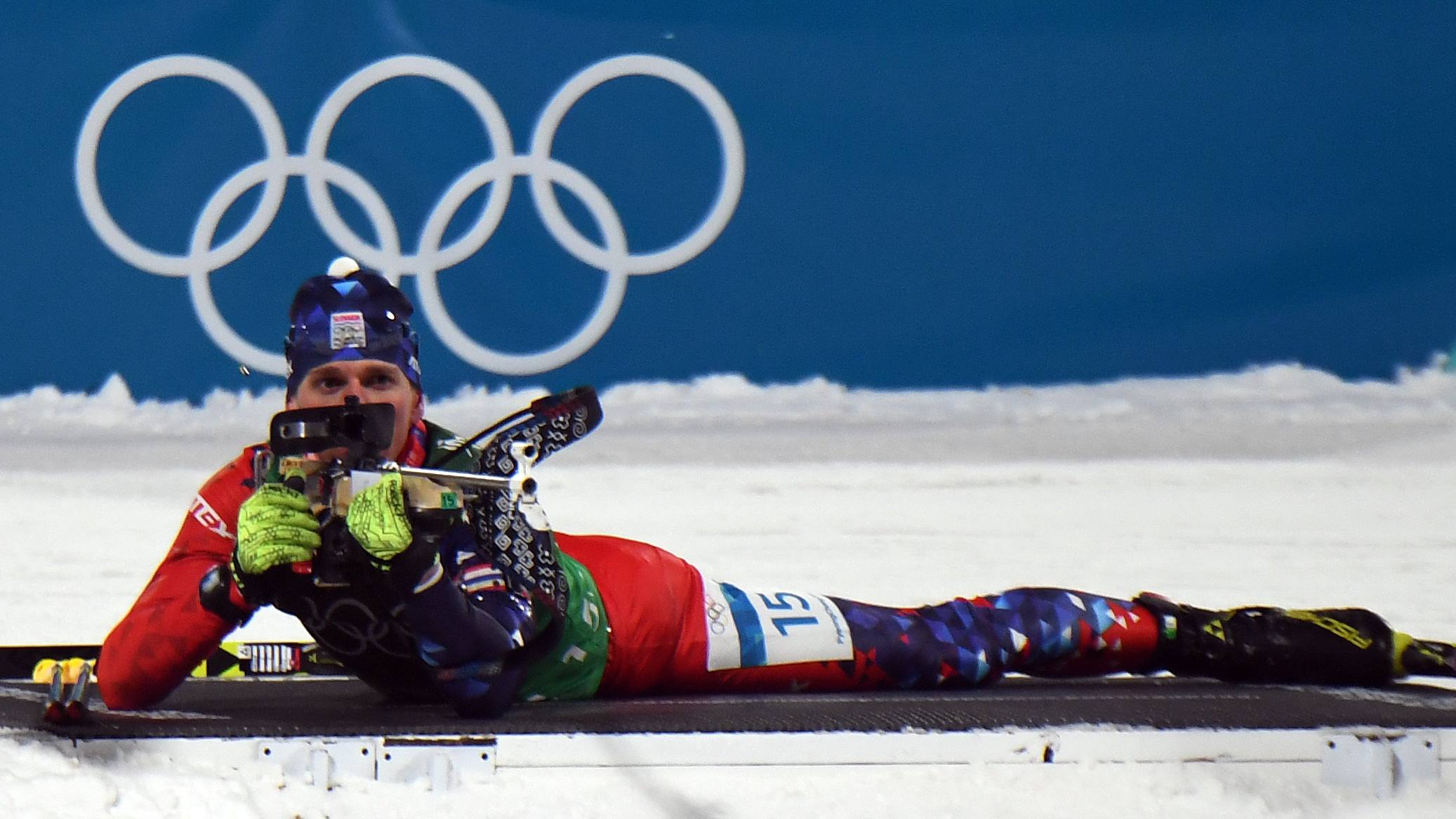The photograph features an Olympic athlete participating in what appears to be a winter shooting sport. The athlete is dressed in a tight-fitting, colorful Olympic outfit incorporating red, green, blue, and white, with yellow gloves and ski boot-like footwear. A beanie and headgear keep him warm, suggesting harsh, snowy conditions. The athlete is lying face down on a black platform, aiming a rifle that features a long silver scope. The gun is poised to shoot, highlighting his intense concentration. Surrounding him, the icy environment reinforces the winter sport setting. Behind the athlete, the iconic Olympic rings are clearly visible on a blue background. The detailed setup and precise gear suggest a highly skilled and focused competitor in an Olympic shooting event.